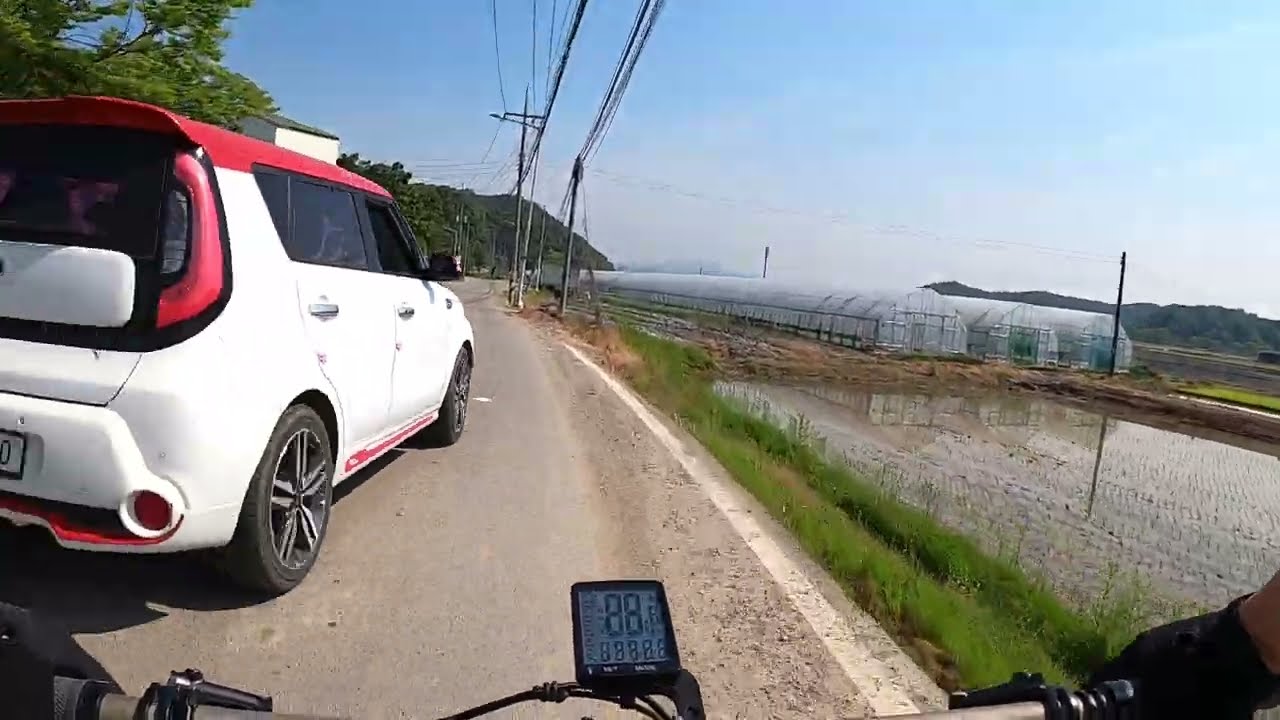A detailed color photograph captured from the perspective of a person on a motorcycle reveals a wide, gray asphalt road. The instrument panel directly in front of the rider features black outlined digital displays, all showing the number 8 in black. The rider's hands are faintly visible gripping the handlebars. Just ahead and to the left of the motorcycle is a white SUV with striking red highlights including a red roof, red lining around the back window, and a red strip at the base between the silver-rimmed tires.

The road is bordered by a white line running along its right side, which becomes more soiled toward the edges. In the vicinity, multiple power lines extend from the center of the road outwards, curving to the left and right. The photograph captures a scenic, countryside landscape. To the far right, long, dome-topped greenhouses stretch into the distance alongside a waterlogged farm, with green vegetation peeking through the water. Further in the background, you can see green hills under a blue sky with scattered white clouds. This idyllic setting gives the impression of a sunny, outdoor adventure, with no other vehicles or buildings immediately nearby, adding to the feeling of solitude and expanse.